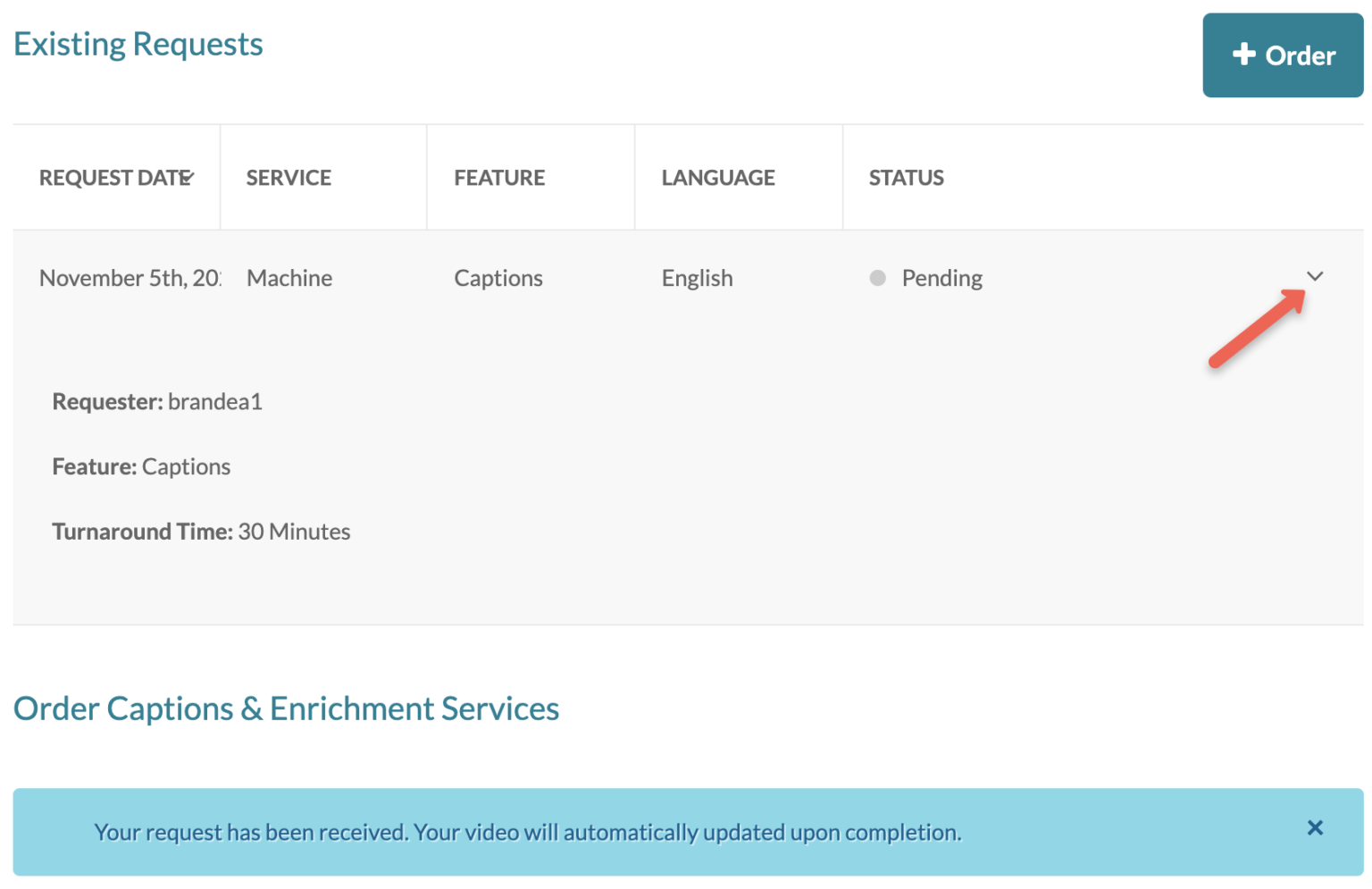This image is a detailed screenshot of an existing requests page, displaying a sleek and minimalist interface with a predominantly white and very light gray background. 

At the top left corner, the page is titled "Existing Requests." On the top right, a prominent blue button labeled "Order" featuring a white plus sign is visible. Below the title "Existing Requests," a horizontal bar lists headings for "Request Date," "Service," "Feature," "Language," and "Status" in that order.

An example entry below these headings shows a detailed breakdown: the request date is November 5th, 20, the service type is "Machine," the feature requested is "Captions," the language is "English," and the status is marked as "Pending." This entry area includes a dropdown menu icon in the upper right corner, highlighted by a red arrow.

Further down, the section labeled "Requester" reveals the requester's name as "Brand EA1." The requested feature is "Captions" with a specified turnaround time of 30 minutes.

At the bottom of the image, a large blue text reads "Order Captions and Enrichment Services." Directly beneath this is a light blue banner that confirms receipt of the request with the message, "Your request has been received. Your video will automatically be updated upon completion." A small blue X at the lower right corner of this footer bar allows users to dismiss this notification.